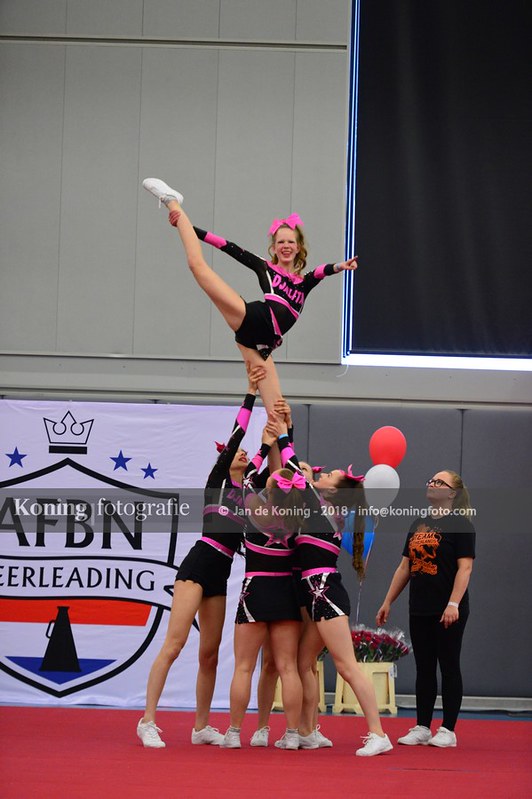In the photorealistic image, we see a striking scene of a cheerleading performance, potentially at a competition. The focus is on four cheerleaders wearing matching black and pink outfits that feature a black skirt with a pink logo and pink bows in their hair. They each sport white shoes. In a coordinated effort, they lift a fifth cheerleader into the air, holding her by one leg extended towards the top left corner of the frame, while she points upwards to the right with a beaming smile on her face. To the right of this dynamic formation, stands a woman with dark hair tied back in a ponytail and dark glasses, dressed in a black shirt with an orange logo and black pants, possibly their coach. The backdrop features a gray wall transitioning to white panels near the ceiling, and prominently displays a white banner with a black crest and the letters "AFBN" along with red and blue designs. The group stands on a red floor, completing the vibrant scene.